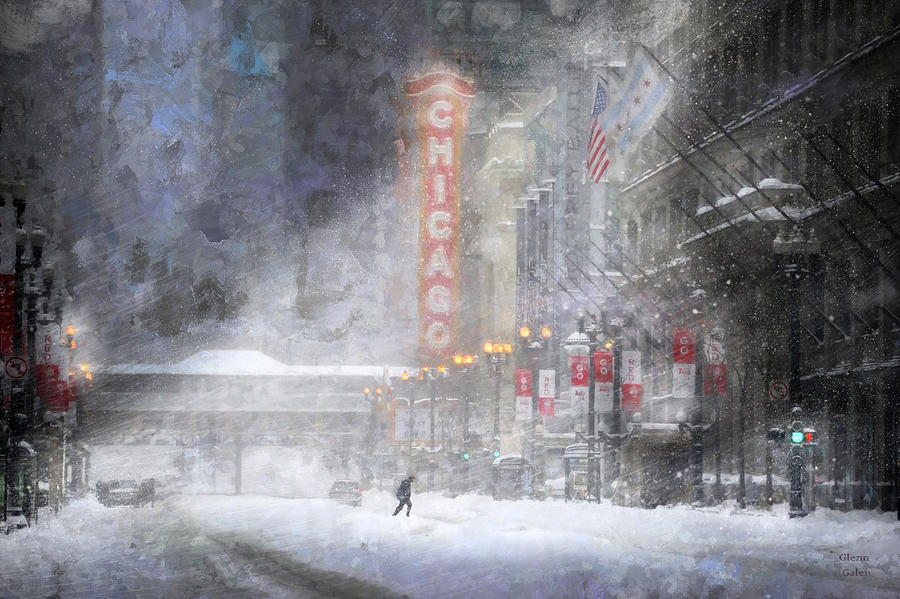The image is an evocative and beautifully muted depiction of a snowy winter street in Chicago, where the atmosphere blurs the line between a drawing and a painting. Captured from the end of the road facing into the city, the scene shows a single thoroughfare with a car approaching the viewer amidst a thick blanket of snow approximately six inches deep. The street is flanked by high buildings on all sides, their gray facades adorned with numerous windows, flags, and streetlights. Prominently, a large vertical red banner with the word "CHICAGO" in bold capital letters stands out, illuminating the center of the image and drawing the eye. On the left side, lights from lampposts and the fronts of buildings provide a warm glow, while on the right, the intricate details of apartment buildings can be seen, complemented by streetlights and yet more flags. A solitary man, dressed in black, is captured mid-crossing, adding a touch of human presence to the tranquil, snowy scene. The bottom right corner of the image features the name "Glenn Gowen" in black lettering.